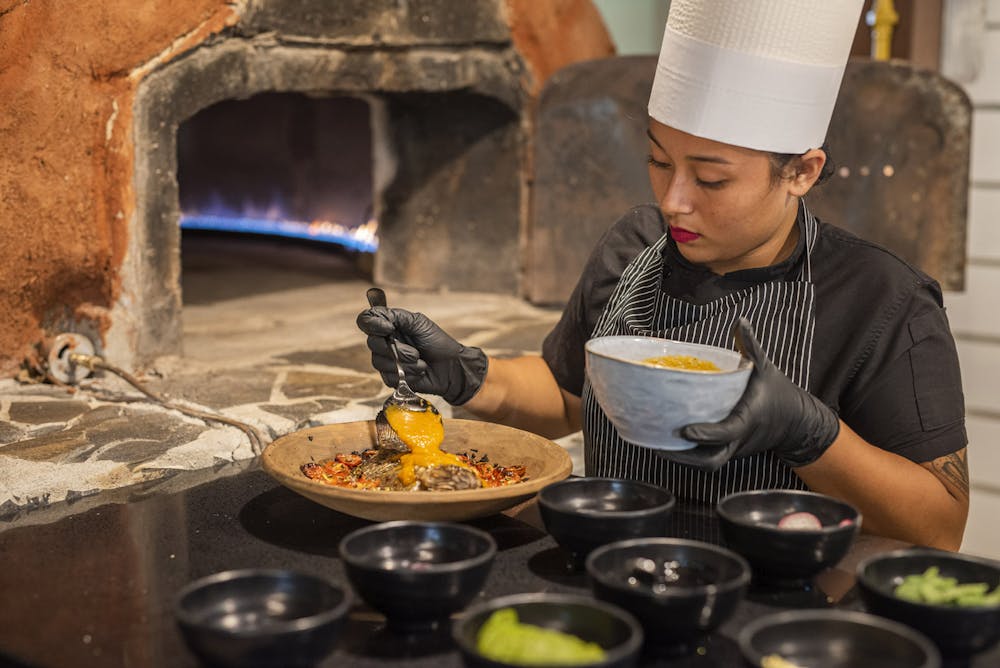In this professionally taken, full-color indoor photograph, a female chef is meticulously preparing a dish at a black countertop laden with numerous black bowls, some containing green ingredients. The chef is attired in a white chef's hat, a white and black striped apron over a black top, and black rubber gloves. A tattoo is visible on her left bicep. She is carefully spooning a yellow cream, which appears to be melted cheese, from a large white bowl into a smaller brown bowl, potentially onto some meat. To her right is a clean, modern gas oven with blue flames, designed to resemble a wood-fire style. The pristine kitchen environment and specialty equipment suggest this is a high-end restaurant. The background features a white wall with some indistinguishable items hanging on it, contributing to the professional and refined ambiance of the kitchen.